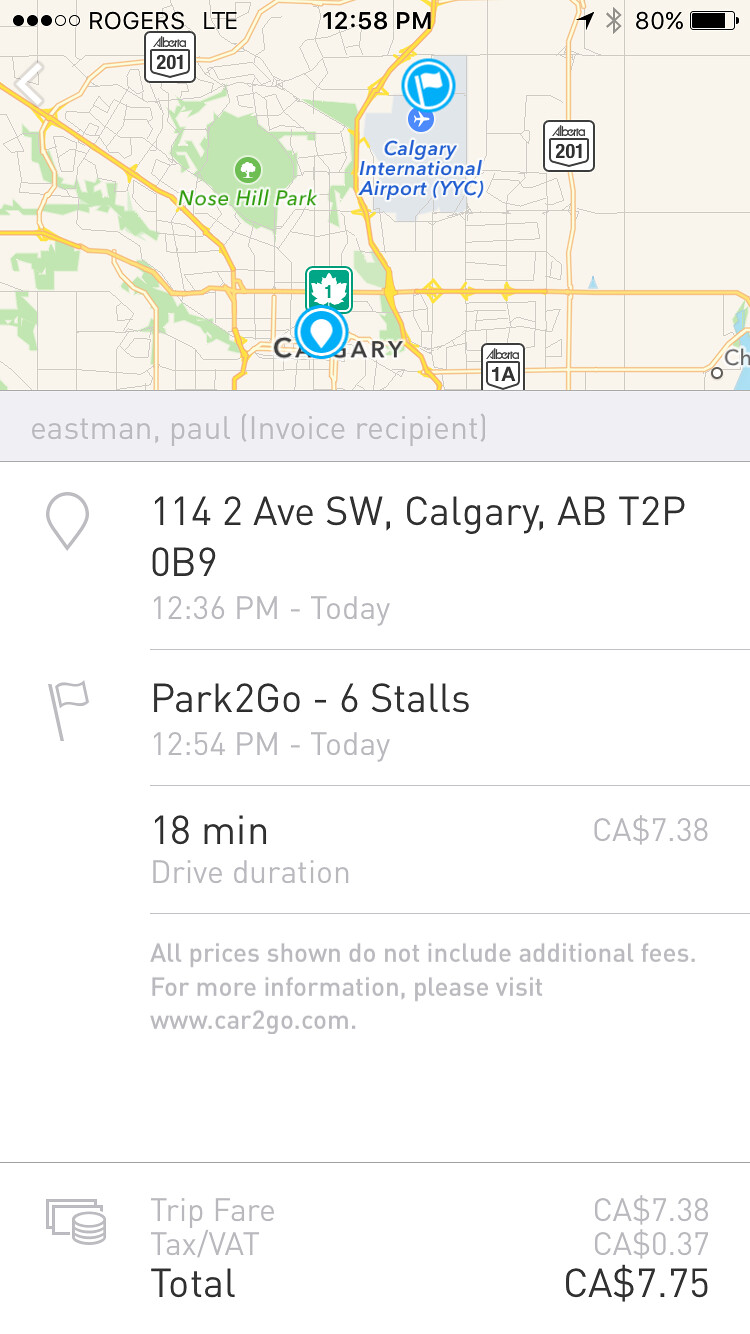The screenshot from a cell phone depicts a Google Maps navigation screen, detailing a route from the user's current location in Southwest Calgary to Calgary International Airport. The top section displays the cell phone's provider as Rogers, the current time at 12:50 p.m., and the battery level at 80%. The map highlights the Calgary International Airport with a blue font and a blue flag icon, while the user's location is marked with a pin labeled as "114.2F SW Calgary AB 2PT 2P OB 9." Below the map, additional information shows Paul Eastman’s name, likely indicating a ride-sharing app interface, along with a message “invoice received.” An image of a parking area labeled "parked to go six stalls" also appears, and the navigation details indicate an 18-minute drive with a cost of $7.38.